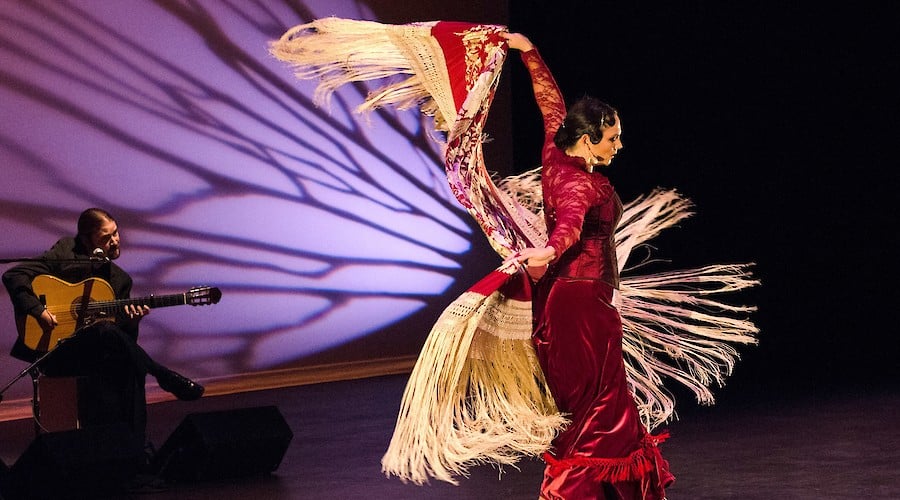In this captivating photograph taken on a dimly lit stage, a talented performer, who appears to be a dancer, takes center stage. She is adorned in an elegant red velvet and lace dress, complemented by a long, ornate shawl in white, red, and floral print with extensive fringe detailing. The dark backdrop of the stage is punctuated by a striking light pattern that resembles butterfly wings, creating an enchanting visual effect. This lighting seems to cast shadows that enhance the ethereal ambiance, making her appear almost butterfly-like as she moves.

In the background to the left, a musician sits on a stool, his leg crossed over the other with an acoustic guitar resting on his lap. He is dressed in an all-black suit and has short brown hair. The microphone positioned near his mouth suggests his readiness to sing, though his head is turned away, indicating he is currently focused on playing. 

The stage floor is either gray or wooden, creating a stark contrast with the light. The walls possess a purple hue, and the side lighting contributes to an almost branch-like cascade effect from the shawl as she manipulates it gracefully. The musician's equipment includes two speakers under his feet, amplifying the music that blends harmoniously with the dancer's performance. Her black hair and fair complexion are subtly highlighted by the soft, ambient light, and a beige headset microphone is visible in her left ear. This detailed setting underscores the synergy between the dancer's fluid movements and the melodious tunes from the guitarist, creating a mesmerizing performance.